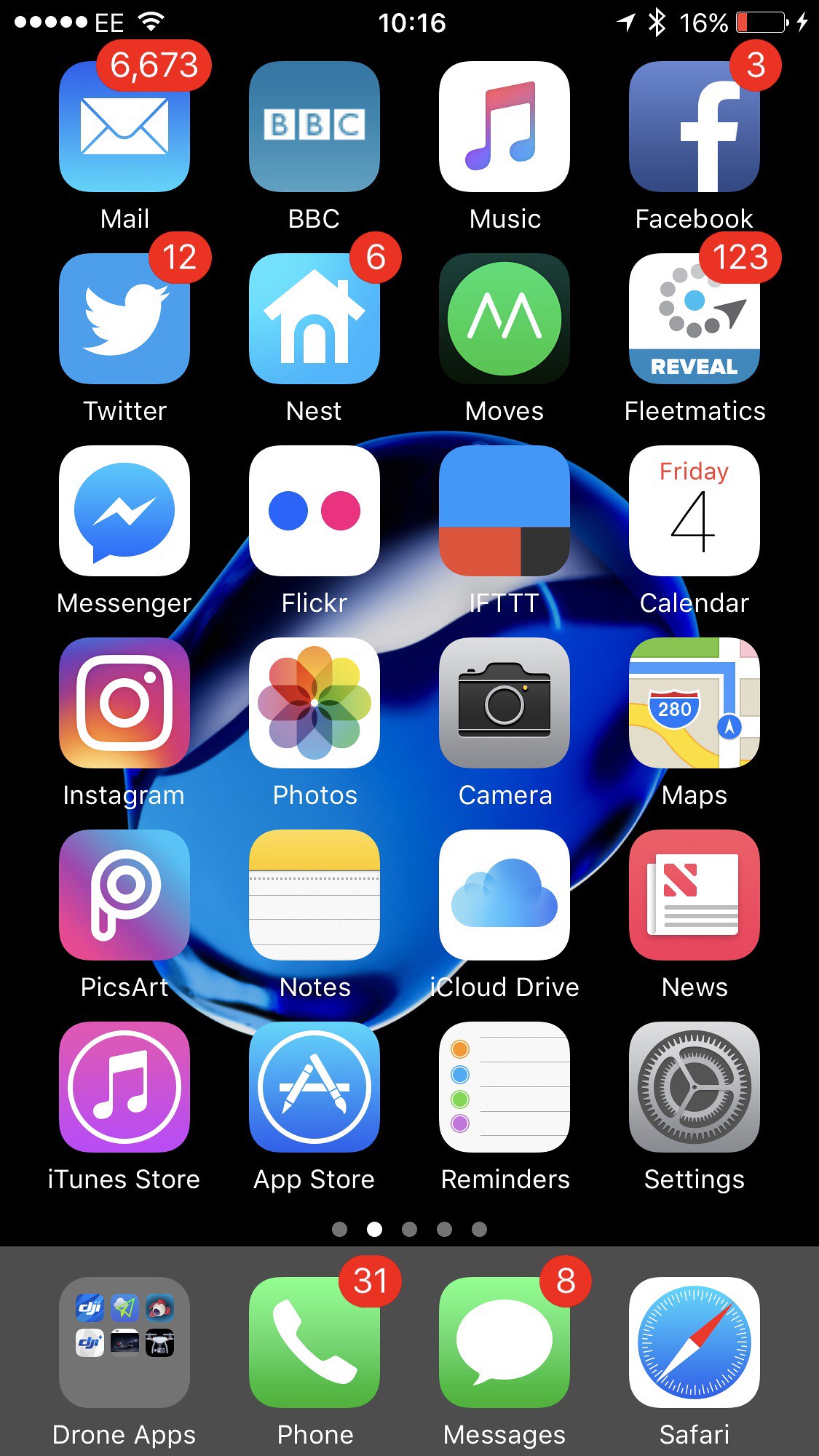This image showcases a smartphone home screen filled with various app icons and notifications. The status bar at the top left features five dots signaling reception strength, followed by the carrier label "EE" and a Wi-Fi symbol in the center. To the right, the time reads 4:16, and the battery is at 16%.

The main screen displays numerous app icons with varying degrees of activity:

Top row:
1. **Mail** - An envelope icon showing 6,673 unread emails.
2. **BBC** - BBC icon positioned next.
3. **Music** - Displayed with a musical note icon.
4. **Facebook** - Represented by a blue "F".
5. **Twitter** - A blue bird icon with a red notification circle showing 12 new notifications.
6. **Nest** - A house icon with six notifications at the top right.

Additional apps:
- **Moose** - Green circle with a white "M".
- **Fleet Maddox** - White icon with a blue accent on the bottom, 123 notifications, and a central blue circle with arrows forming a loop.
- **Messenger** - Standard messaging icon.
- **Flickr** - Blue and pink dots.
- **IFTTT** - Blue square with a small red rectangle in the bottom left corner.
- **Calendar** - Displays "Friday, 4".
- **Instagram** - Rainbow-colored flower icon.
- **Camera** - Minimalistic camera icon.
- **Maps** - Traditional maps icon.
- **Pixar** - A blue circle with a "P" inside.
- **Notes** - White note icon with a yellow top.
- **iCloud Drive** - White square with a light blue cloud.
- **News** - A newspaper icon on a red background.
- **iTunes Store** - Purple circle with a music note.
- **App Store** - Blue square with a white "A".
- **Reminders** - Icon showing multicolored bullet points: orange, blue, green, and purple.
- **Settings** - Gear icon, slightly iterated.

The dock at the bottom includes:
1. **Phone** - Green square with a phone icon, indicating 31 notifications.
2. **Messages** - Green square with a white speech bubble.
3. **Safari** - Compass icon with North pointing to the upper right and South to the lower left.

The screen offers an in-depth snapshot of a highly used smartphone, cluttered with various app notifications and easily recognized icons, representing a user's daily digital interactions.